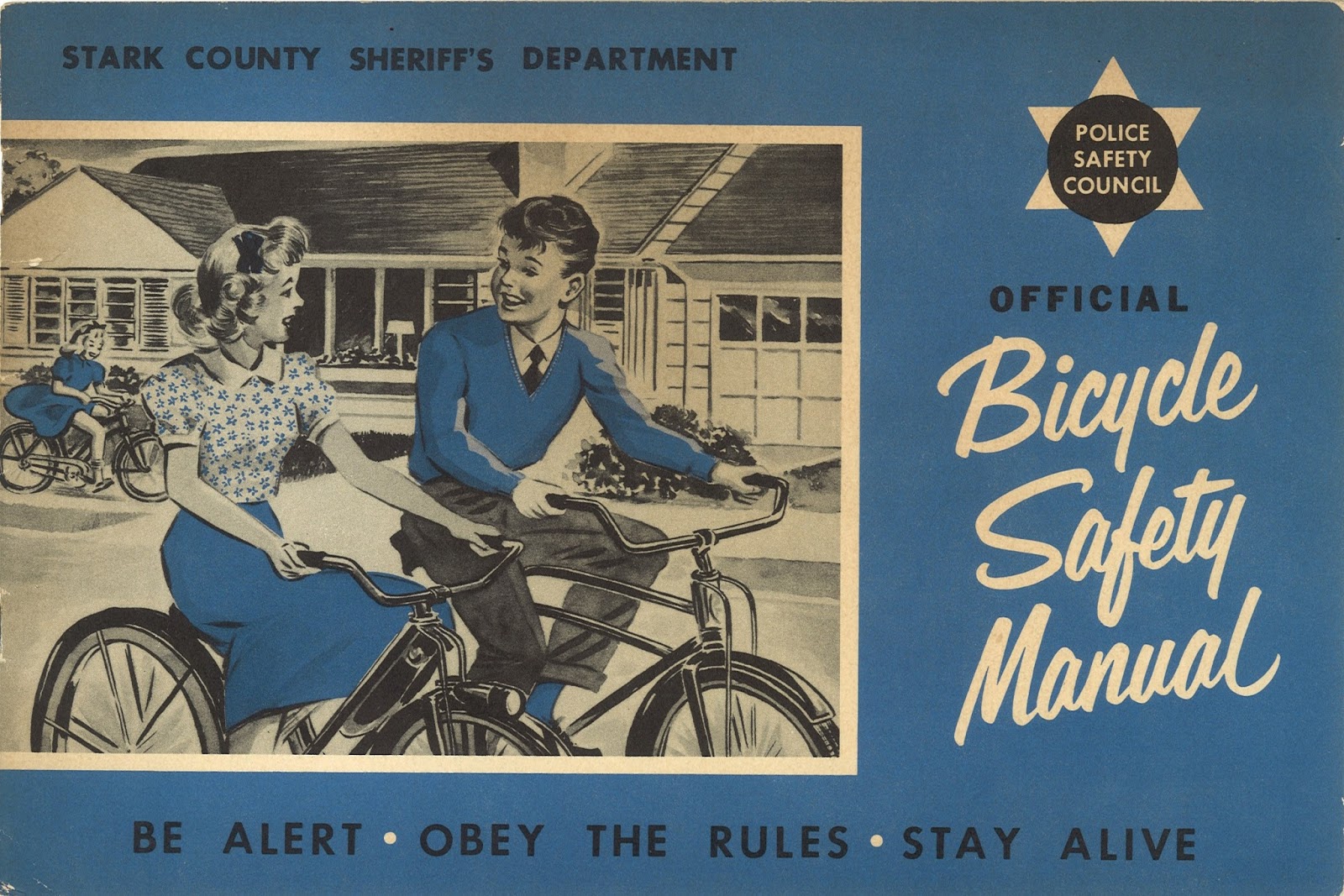This image is a vintage cover of a bicycle safety manual from the 1940s or 1950s, produced by the Stark County Sheriff's Department in association with the Police Safety Council. The background is predominantly a dull blue, with all text in dark blue, black, or white. The manual prominently features the safety admonitions: "Be alert. Obey the rules. Stay alive."

The scene is reminiscent of classic mid-20th century America, akin to the idyllic settings of "Donna Reed" or "Leave it to Beaver." It depicts three children riding bicycles against the backdrop of a monochromatic, ranch-style home typical of the era. The illustration is partially colored, using shades of blue consistently across the children’s clothing. 

In the foreground, a boy dressed in black trousers, a blue sweater over a white shirt, and a black tie rides alongside a girl wearing a blue skirt and a blue-and-white printed blouse. Both children are interacting cheerfully. A third child, a girl in a blue dress, rides her bike on the sidewalk further in the background. Behind them, the house features a picture window revealing a lamp and a garage with square windows. The composition emphasizes a safe and attentive approach to bicycling, reinforcing the manual’s purpose.